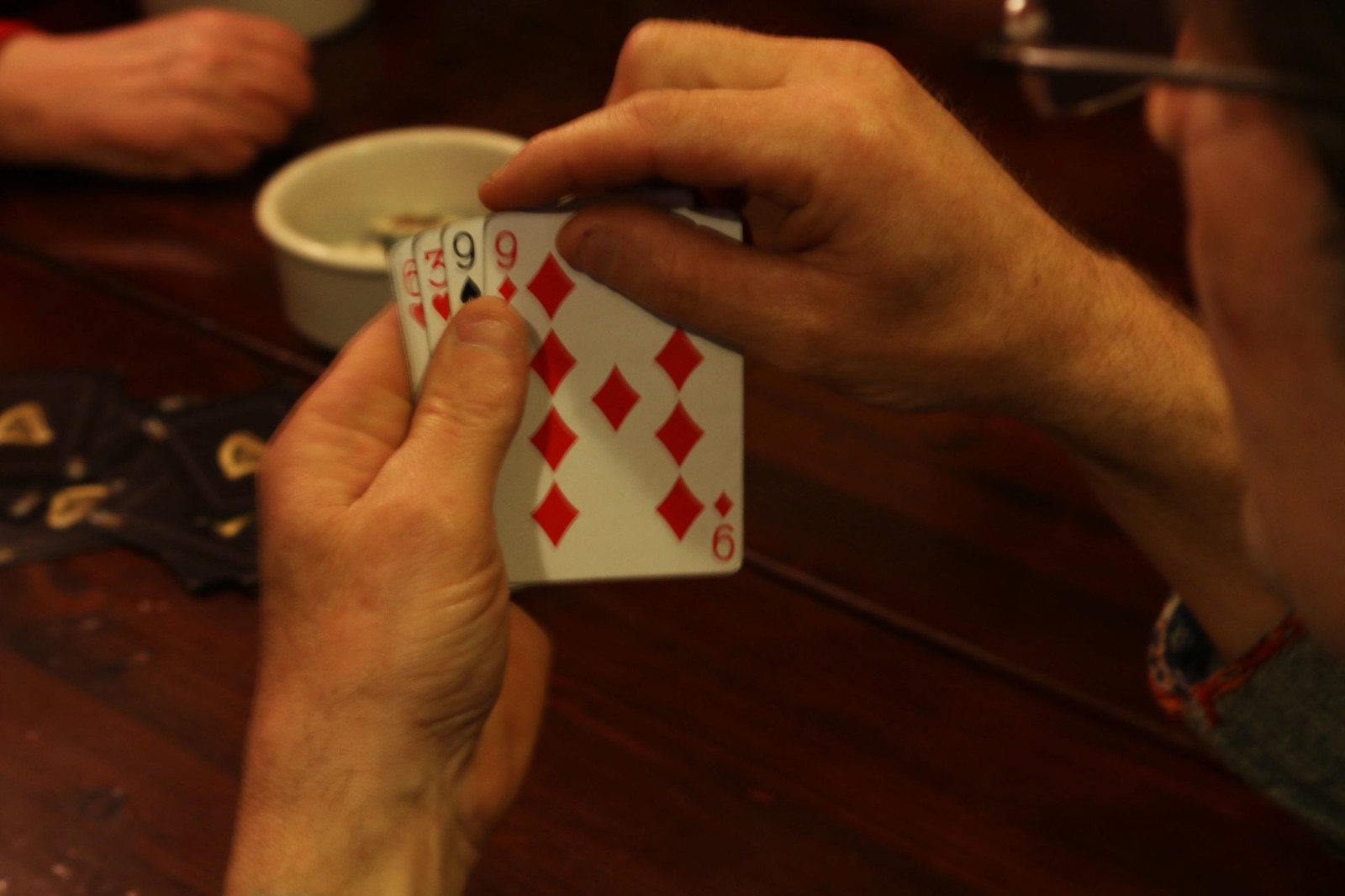This horizontal image captures an intimate indoor scene with a warm, yellow-orange cast due to natural low light. At an unknown location, a white gentleman is prominently featured, viewed from the waist up, with the focal point being his hand of playing cards. He wears glasses and a long-sleeve shirt, and his left wrist appears to be adorned with a watch. He is holding four playing cards in his left hand, with his right hand gently resting on the top cards, which are the nine of diamonds, nine of spades, three of hearts, and six of hearts, revealing a pair of nines. The setting suggests a casual game, indicated by dimly visible dark objects, possibly poker chips, on the table behind him. A white bowl sits above these objects, hinting at snacks or game accessories. In the upper left corner, the hand of another player, also a white gentleman, emerges into the frame, adding depth to the composition. The image's overall ambiance is somewhat dark and slightly blurry, contributing to its candid and cozy atmosphere.